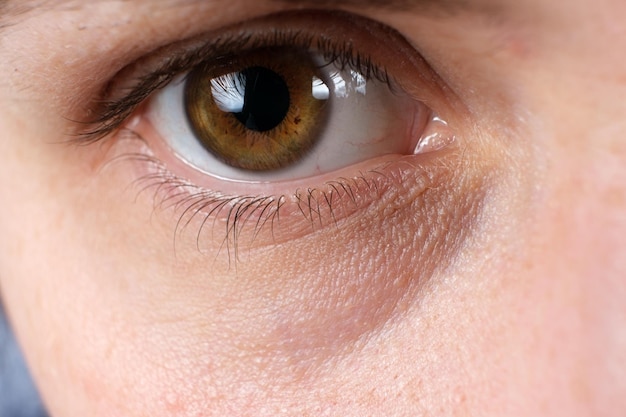The photograph is a highly detailed close-up of a person's eye in a landscape layout, where the width is short compared to the height. The subject's eye is predominantly hazel, with nuanced shades of green, brown, and a golden amber hue near the center. The black pupil is prominent, taking up a significant portion of the eye. The surrounding sclera is exceptionally clear, devoid of redness. Visible are well-groomed dark brown eyelashes and a light brown eyebrow in the upper left corner. The image captures not just the eye but also extends to show part of the bridge of the nose, a tiny hint of the cheek, and a slight skin wrinkle under the eye. The background in the lower left-hand corner features a bluish-gray color. The person's Caucasian skin is evident, but the minimal visible facial features make it difficult to determine age or gender. Reflections of light on the eye suggest either natural room lighting or a camera flash.